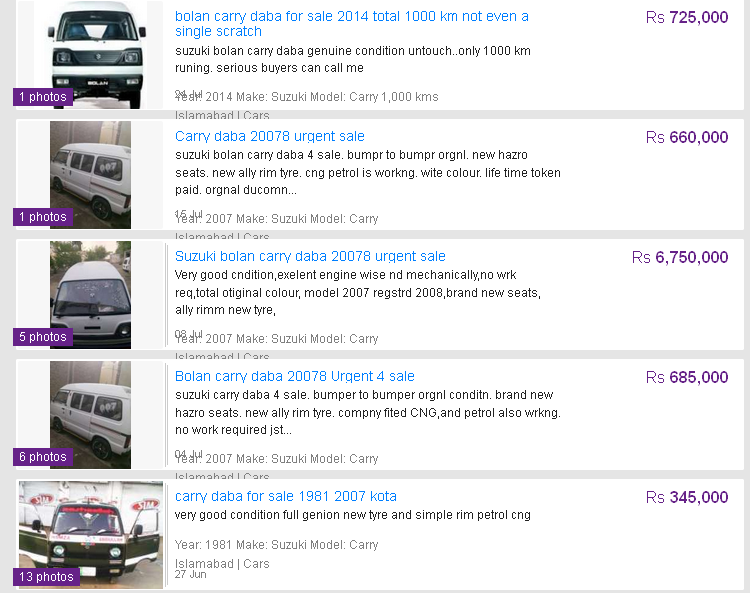**Detailed Vehicle Listings on Aggregated Website Similar to Craigslist for Cars**

**Left Section:**

- **White Van Listing**:
  - Title: **Mullen Carry DABA for Sale**
  - Year: **2014**
  - Mileage: **1000 KM**
  - Condition: **Not a Single Scratch**
  - Price: **RS725** (South African currency)
  - Description: **Suzuki Bullen Carry DABA, genuine condition, untouched with only 1000 KM running. Serious buyers can call me.**
  - Model Details: **2014 Suzuki Carry with 1000 KM.**
  - Image: **Side view of a white van**
  - Hyperlink: **Carry DABA 20078 Urgent Sale**

**Right Section:**

- **White Van Comprehensive Details**:
  - Title: **Suzuki Bullen Carry DABA for Sale**
  - Year: **2007**
  - Mileage: **1000 KM**
  - Description: **BUMPR to BUMPR original condition. New HAZO seats, new ALIRIM tires, CNG and petrol working, white color, lifetime token paid, original DUCOMN.**
  - Price: **RS660,000**
  - Model Details: **2007 Suzuki Carry**
  - Condition: **Very good, excellent engine and mechanically sound, no work required, total original color. Registered 2017. Brand new seats, new ALIRIM type.**
  - Image: **Front view of another white van**
  - Hyperlink: **Suzuki Bullen DABA 20078 Urgent Sale**
  
- **Another Listing for Similar Vehicle**:
  - Title: **Bullen Carry DABA Urgent Sale**
  - Year: **2007**
  - Condition: **BUMPR to BUMPR original condition, company fitted CNG and petrol also working, no work required, just perfect.**
  - Price: **RS6,750,000**
  - Model Details: **2007 Suzuki Carry**
  - Image: **Side photo of the van**
  - Hyperlink: **Bullen Carry DABA 20078 Urgent Sale**

- **Black Van Listing**:
  - Title: **Carry DABA for Sale**
  - Year: **1981**
  - Price: **RS345,000**
  - Condition: **Full genuine, new tire in simple rim, petrol, and CNG.**
  - Model Details: **1981 Suzuki Carry**
  - Location: **Islamabad**
  - Hyperlink: **KOTA 20078 Urgent Sale**

**Summary**: These listings appear to feature multiple instances of Suzuki Bullen Carry DABA vans, predominantly from 2007 and 2014, all in varied states of excellent condition and sporting new updates such as seats and tires. They are marketed towards serious buyers, with specific details on mileage, mechanical condition, and urgency of sale. The black van in 1981 model offers a bargain price with similar genuine conditions and is located in Islamabad.